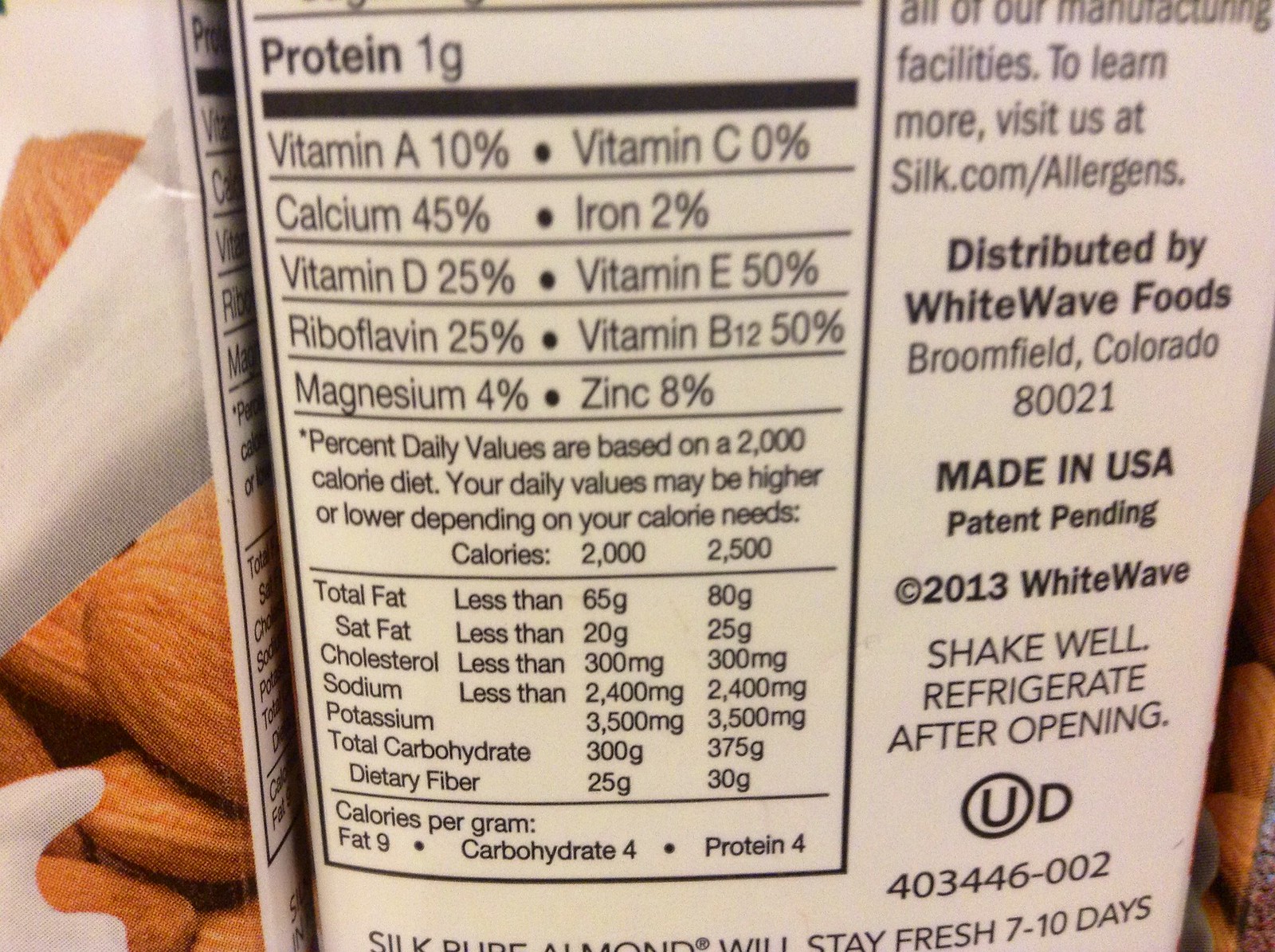This vibrant color photograph captures a meticulously detailed close-up view of a carton of Silk Pure Almond almond milk. The label, which is featured prominently, reveals an extensive section of nutritional information. At the top, it mentions "Protein 1 gram" and includes percentages of daily values for vitamins and minerals, such as 45% of calcium, 10% of vitamin C, and 2% of iron. The background image combines almonds with a cascading stream of milk. To the left, another carton of almond milk is positioned sideways, showcasing the artwork of almonds and milk pouring, while a sliver of yet another carton peeks from the right. The text on the carton includes details about the product, stating "Distributed by White Wave Foods, Broomfield, Colorado," along with the instructions "Shake well, refrigerate after opening." Additional clear notations include "Made in USA" and "patent pending" in bold. Furthermore, at the bottom of the carton, it is stated that "Silk Pure Almond will stay fresh for 7 to 10 days."